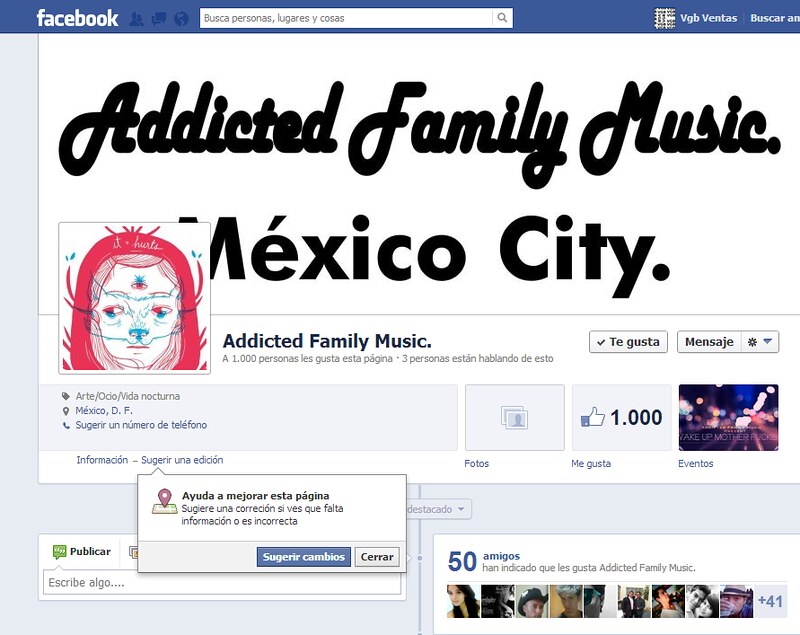This screenshot captures a nostalgically designed Facebook page from an older version of the platform, headlined with "Addicted Family Music" and "Mexico City" prominently displayed in bold fonts. At the top, there's a blue horizontal band featuring the classic Facebook logo, a search bar that reads "Buesca Personas Lugares y Cosas," and other navigational aids. 

To the left, the profile picture is a surreal, sketch-style illustration of a three-eyed person clad in a pink (or red) hoodie with red swaths of hair. The figure has a dog-like nose, regular lips, and a sketchy outline resembling a mask around their eyes, sparing the central third eye. The banner indicates 1,000 likes, and there's a prominent "50 Amigos" below it, indicating the profile has 50 friends, visually supported by a grid showing 9 friends and a "+41" label. The user has shown engagement with other pages, such as "Aventos" and "Mi Gusta." The lower section of the page features options to view photos and other interactions. The image prominently captures the vintage Facebook aesthetic with its distinct color blocks and retro fonts.